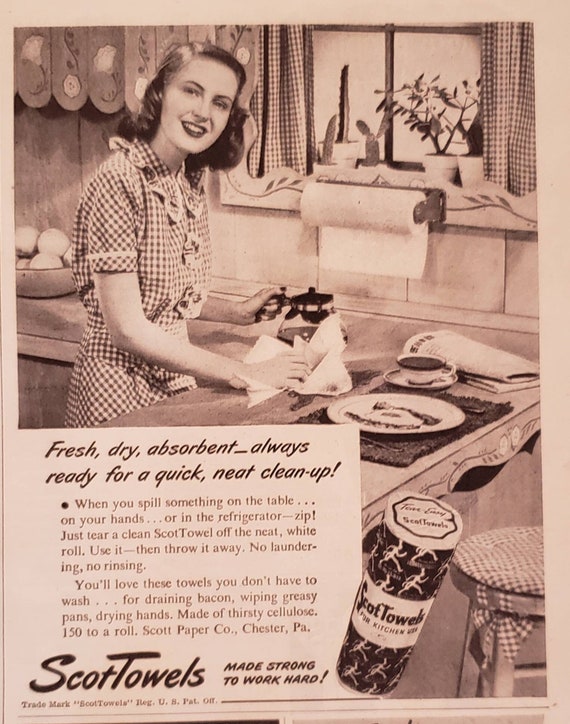This vintage advertisement from the 1950s or 1960s for Scott Towels, featuring the slogan "Made Strong to Work Hard," showcases an era-specific scene detailed with precision. The ad is on a pinkish paper with a decorative border on the top and right side, and a thin border on the left. In the upper left corner, a black and white image of a woman dressed in an old-fashioned, polka-dot dress suggests the ad's age. Her shoulder-length dark hair frames her face as she glances back while cleaning up a spill. Her right hand holds a white paper towel on the counter, and her left hand grips the handle of a coffee pot. The counter extends from the foreground to behind her, curving to her right. A roll of paper towels is mounted below a window adorned with small potted plants and polka-dotted curtains. 

To the right of the woman, on the counter, there is a plate on a placemat accompanied by a cup of coffee and a newspaper. A stool with a polka dot seat and wooden legs appears to the far right. The text in the bottom left gray box states, "Fresh, dry, absorbent, always. Ready for a quick, neat clean-up." The ad further highlights the convenience of the product with detailed instructions, "When you spill something on the table, on your hands, or in your refrigerator, just tear a clean Scott Towel off the neat white roll. Use it, then throw it away. No laundering. No rinsing. You'll love these towels. You don't have to wash for draining bacon, wiping greasy pans, drying hands. Made of thirsty cellulose, 150 to a roll." 

The advertisement concludes with the brand details prominently displayed: "Scott Towels, made strong to work hard," along with the company name, Scott Paper Company, Chester, Pennsylvania, solidifying its legacy with the trademark information, "Scott Towels, Reg US Pat off."